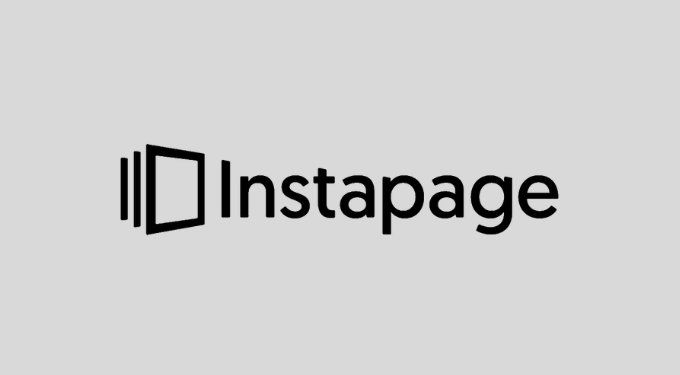The image depicts a landscape-oriented photograph, approximately 1.5 to 2 times wider than it is tall, featuring the logo of a company named "Instapage." The background of the image is a monochromatic gray, providing a neutral canvas for the centrally aligned elements. Dominating the center of the image is the word "Instapage," presented in a sleek, black font that is perfectly centered both vertically and horizontally.

To the left of the "Instapage" text, there is a distinctive logo. The logo comprises three elements arranged sequentially: a short vertical line on the left, a slightly taller vertical line to its right, and finally, an angled square. This square appears to be rotated, contributing to the overall sense of depth and dimension. The interior of the square is gray, while its border is black, harmonizing with the "Instapage" text. The logo's design conveys a subtle 3D effect, enhancing its visual interest.

The image does not include any additional text, images, or contextual information about the company. Although the viewer might speculate that Instapage could be related to technology or social media, resembling other well-known platforms, the image itself provides no further clues about the nature or services of the company.